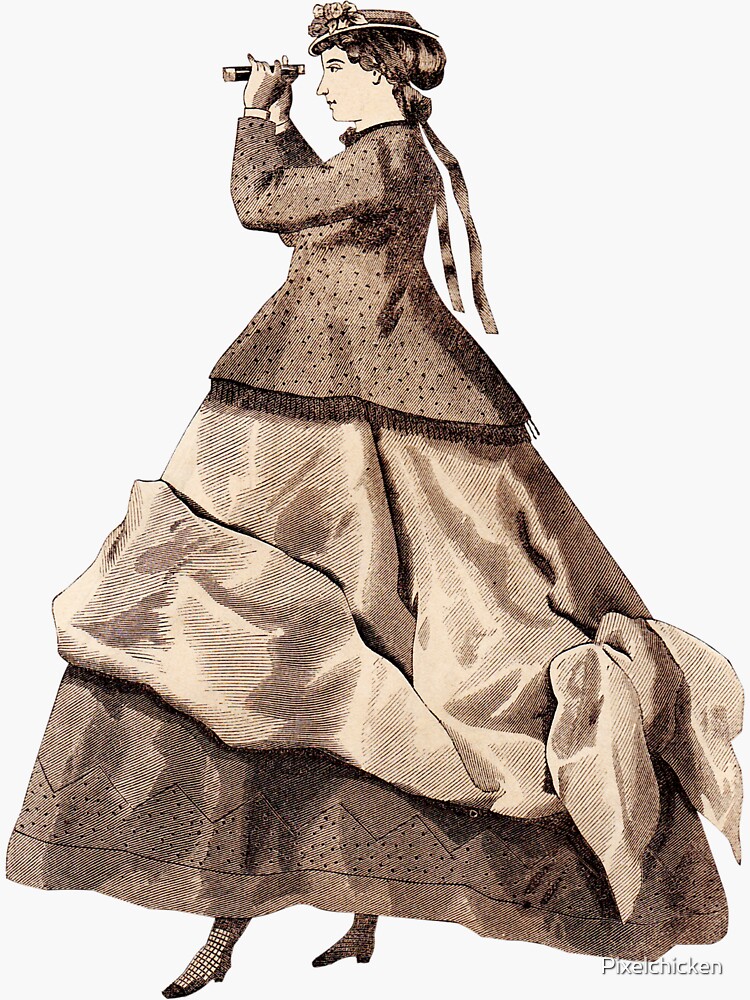The image depicts a detailed painting of a woman viewed from the side, facing left. She is an old-fashioned figure with her hair pulled back in a bun and secured by ribbons that dangle down to her waist. The woman wears a large, heavy tan and brown dress or overcoat, possibly made of wool, that widens towards the bottom and features a frilled skirt. A spotted waistcoat adds to her elaborate attire. A sun hat or bonnet with ribbons hangs from her head, and she dons shoes with visible socks or stockings. In her hands, she holds a pair of binoculars, which she is looking into. The painting has a white background and is vertically oriented. At the bottom right of the painting, the text "pixel chicken" is visible.